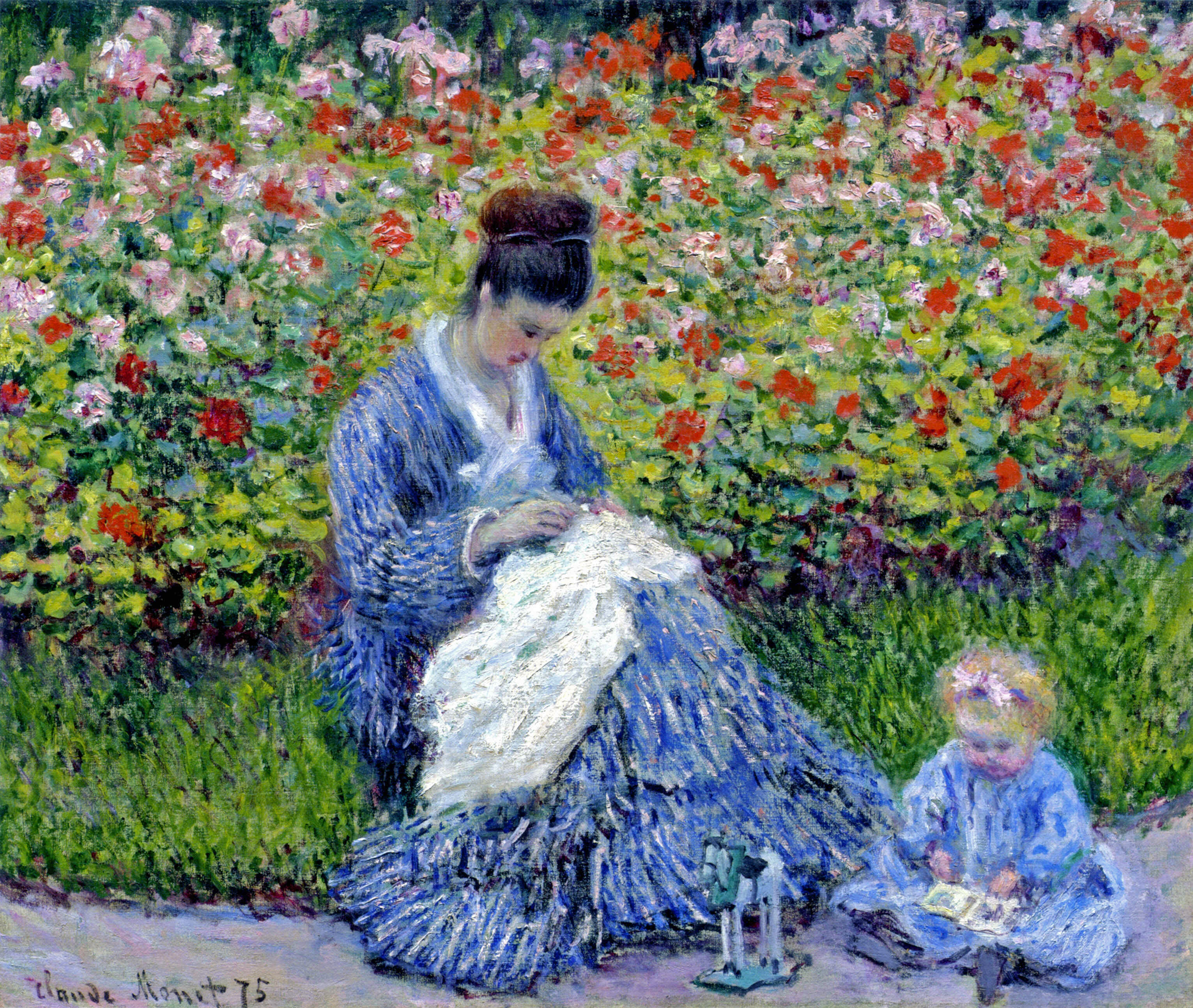In this vibrant, impressionistic painting by Claude Monet, dated '75, a white woman with dark hair styled in an updo is depicted sitting on a patch of lush green grass. She is adorned in a long, ruffled blue dress, diligently sewing a piece of white material that rests in her lap. Beside her, a small blonde-haired girl, possibly her daughter, sits on the ground wearing a similar blue dress with a pink headband. The little girl appears engrossed in reading a book, with a white toy horse, accented with green, lying nearby. The background is filled with an explosion of colorful flowers in shades of red, pink, white, and hints of purple, encapsulating a lively summer or spring outdoor setting. The painting exudes a sense of warmth, light, and the tranquil beauty of nature.